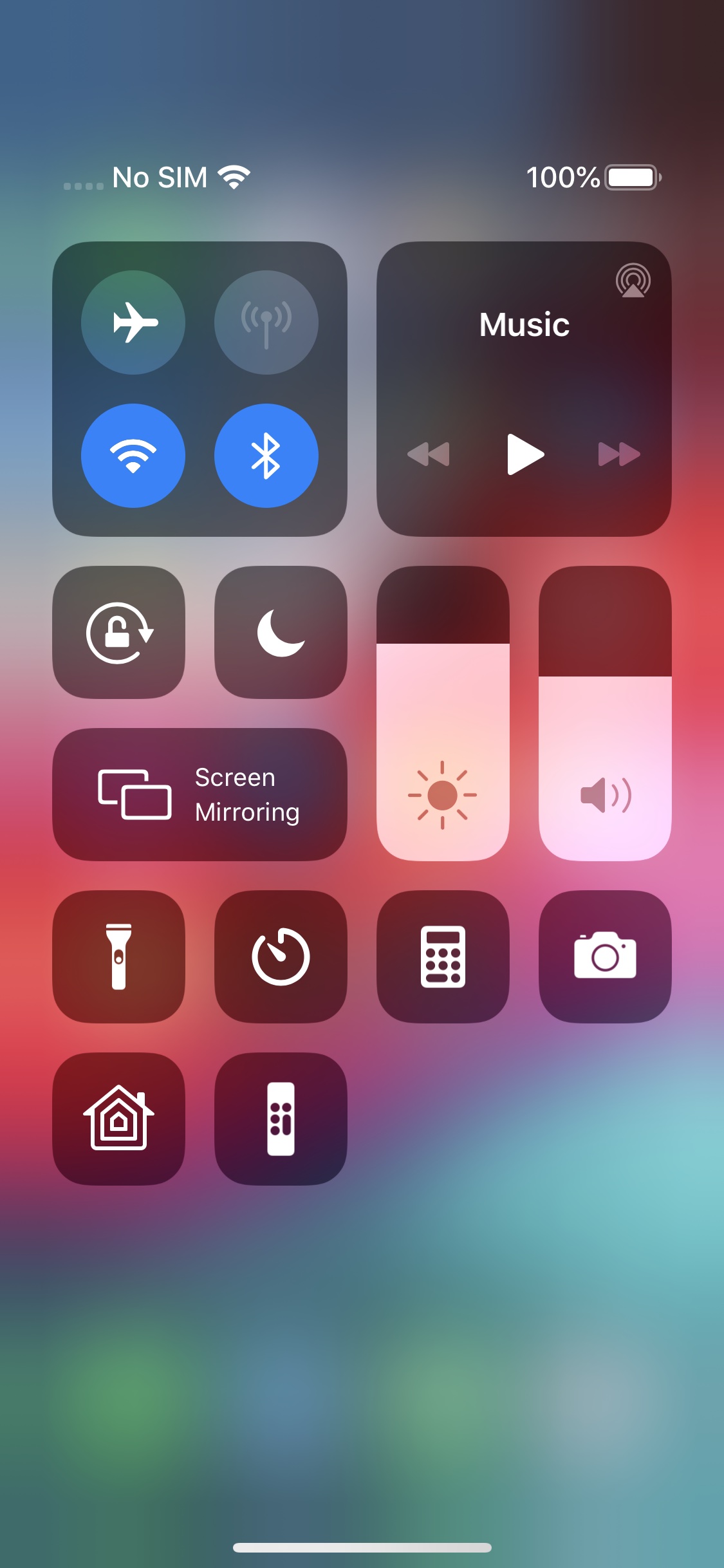The image showcases the Notification Center of an iPhone, an Apple iOS device. The background displays a slightly glaring wallpaper with a gradient of colors. At the bottom, the wallpaper features a blend of purple and green hues. The center area is dominated by a pink shade, and towards the top, dark tones are interspersed with light blue colors.

On the left side of the Notification Center, several toggles and icons are visible: 
- Airplane Mode 
- Hotspot 
- Bluetooth (highlighted in blue indicating it is active) 
- Wi-Fi (also highlighted in blue indicating it is active) 
- Rotation Lock 
- Night Mode 
- Screen Mirroring 
- Light Switch 
- Timer/Clock 
- Home System Switch 
- Remote Switch (likely for Apple TV or similar devices)

On the top right, there is a music player widget with controls for play, preview, rewind, and forward. Below this, a brightness slider almost at its maximum level, shaded in white against a gray background, is visible. Further down, there is a volume slider positioned approximately in the middle of its range. Towards the bottom right, white icons for Calculator and Camera are also present.